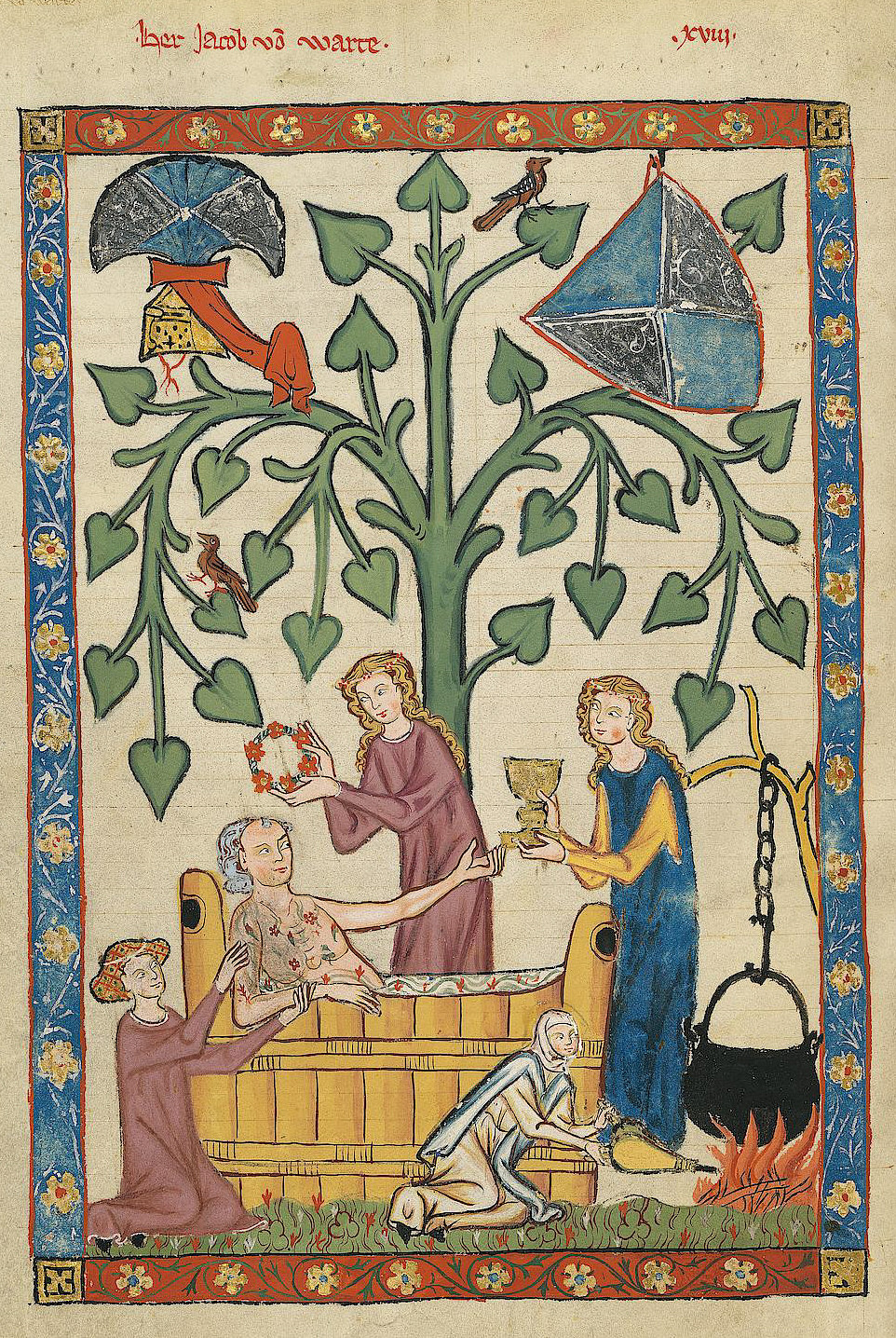The image is a detailed, medieval-style illustration depicting a wealthy man in a wooden bathtub with a backrest and an elevated footrest, each featuring a black circular design. The man, who appears injured or burnt, is attended by several peasant women. One woman in a red gown and a flower headband is placing a wreath on his head, standing just behind him. Another peasant woman, dressed in a red dress, is rubbing his injured side, while a third woman, wearing a blue gown with yellow sleeves, offers him a brass cup from the foot of the tub. Kneeling near the bottom left of the tub, a woman in a maroon robe tends to one of his arms. 

In the background, a green tree with heart-shaped leaves and red birds spreads its branches across the image. Near the bottom right corner, a peasant woman fans a fire beneath a large black kettle hanging from a tree limb. The edges of the illustration are intricately bordered: the top and bottom with red and white flowers, and the sides with blue and floral designs, each corner adorned with a gold square. At the top, there is red writing in a foreign language. A shield and another brass object with a blue and black fan and a red ribbon can also be spotted within the scene.